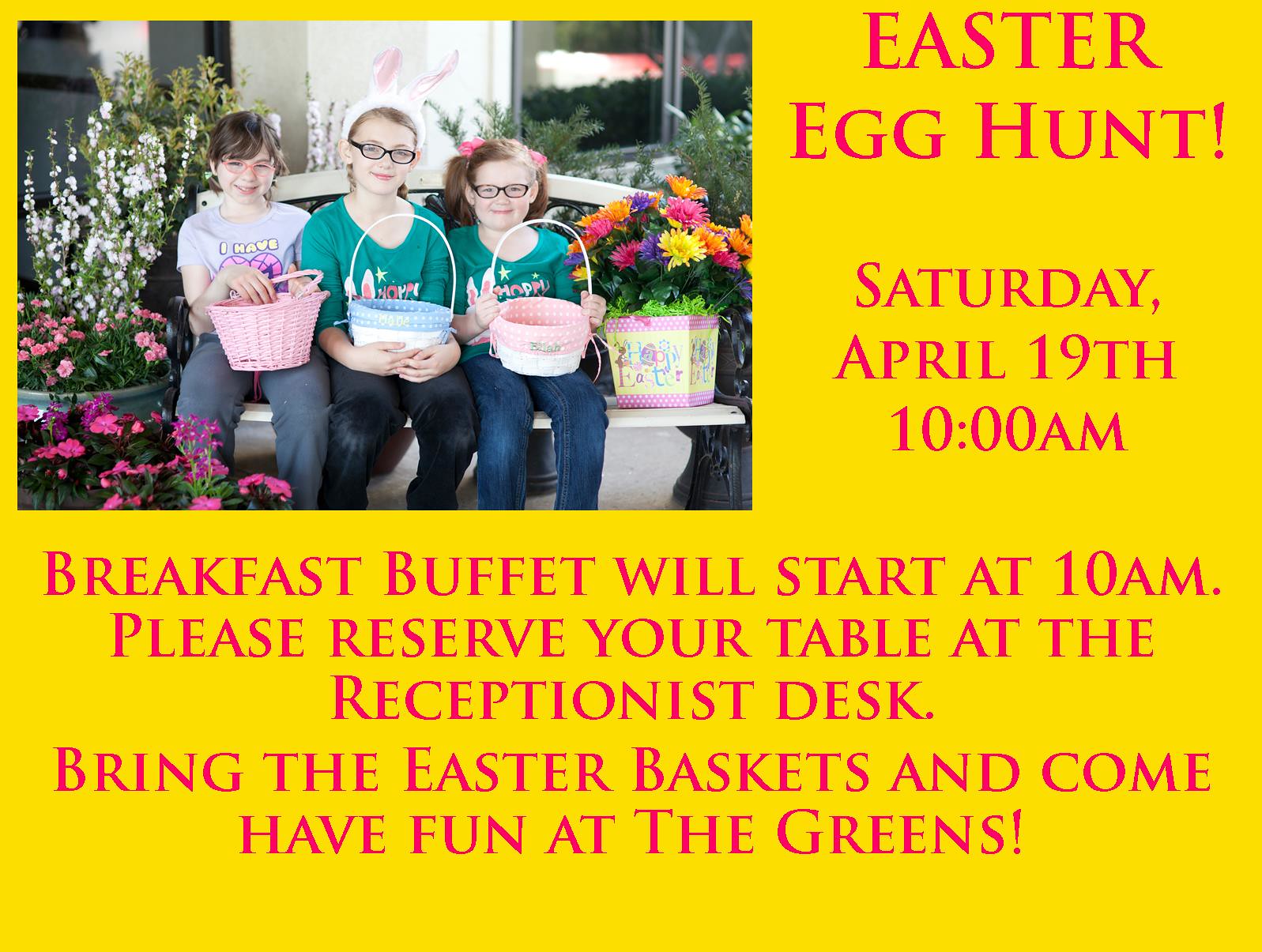This vibrant poster advertises an Easter egg hunt and prominently features a photo in the top left corner of three young children sitting on a white concrete bench, all holding Easter baskets in their laps. The two children on the right wear green t-shirts and glasses, while the child on the left wears a light blue shirt and also has glasses. The center child dons bunny ears. Colorful flowers surround the children, adding a festive touch, including a square pot on the right side containing pink, purple, yellow, and orange flowers, decorated with Easter eggs. The poster’s background is yellow, with pink letters that read: "Easter Egg Hunt, Saturday, April 19th at 10 a.m." Below this text, it mentions a "Breakfast Buffet will start at 10 a.m. Please reserve your table at the receptionist's desk," and "Bring Easter baskets and come have fun at the Greens." This image is set in an outdoor ambiance, possibly with a building and windows visible in the background.